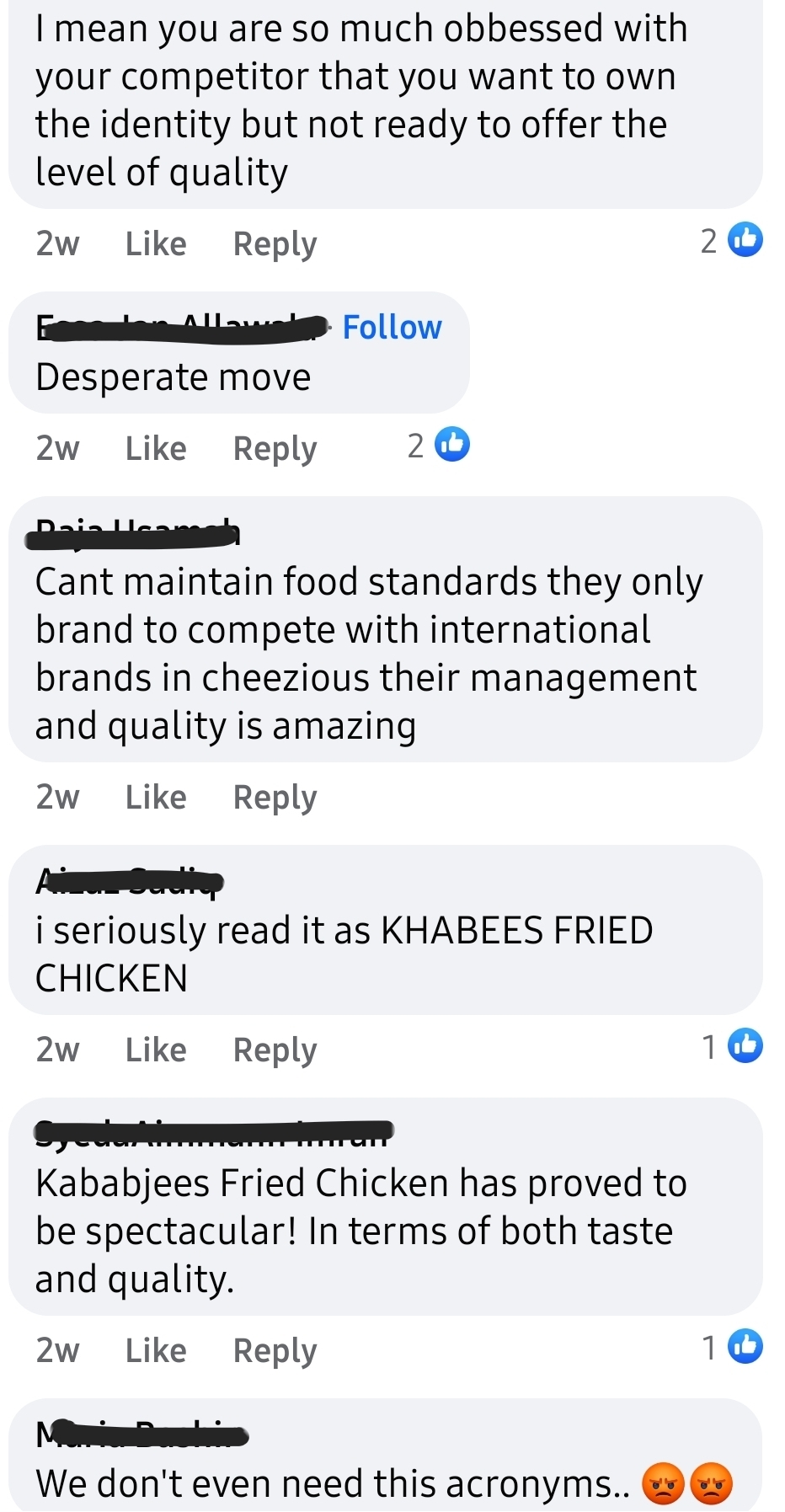The image depicts a conversation encapsulated in gray boxes, each containing a timestamp, a like button, and a reply button, along with a visual tally of the number of thumbs-up received for that comment. 

The top comment reads, "I mean, you are so much obsessed with your competitor that you want to own the identity, but you are not ready to offer the level of quality," reflecting a critical view on competitive behavior and quality standards. 

The second comment is partially redacted and succinctly states, "Desperate move."

The third comment, with the commentator's name redacted, opines, "Can't maintain food standards. They only brand to compete with international brands. Cheesiest. Their management and quality is amazing," highlighting both criticism and admiration within the same breath.

The final comment in the thread humorously reads, "I seriously read it as kibibs fried chicken," suggesting a playful misunderstanding of a brand's name.